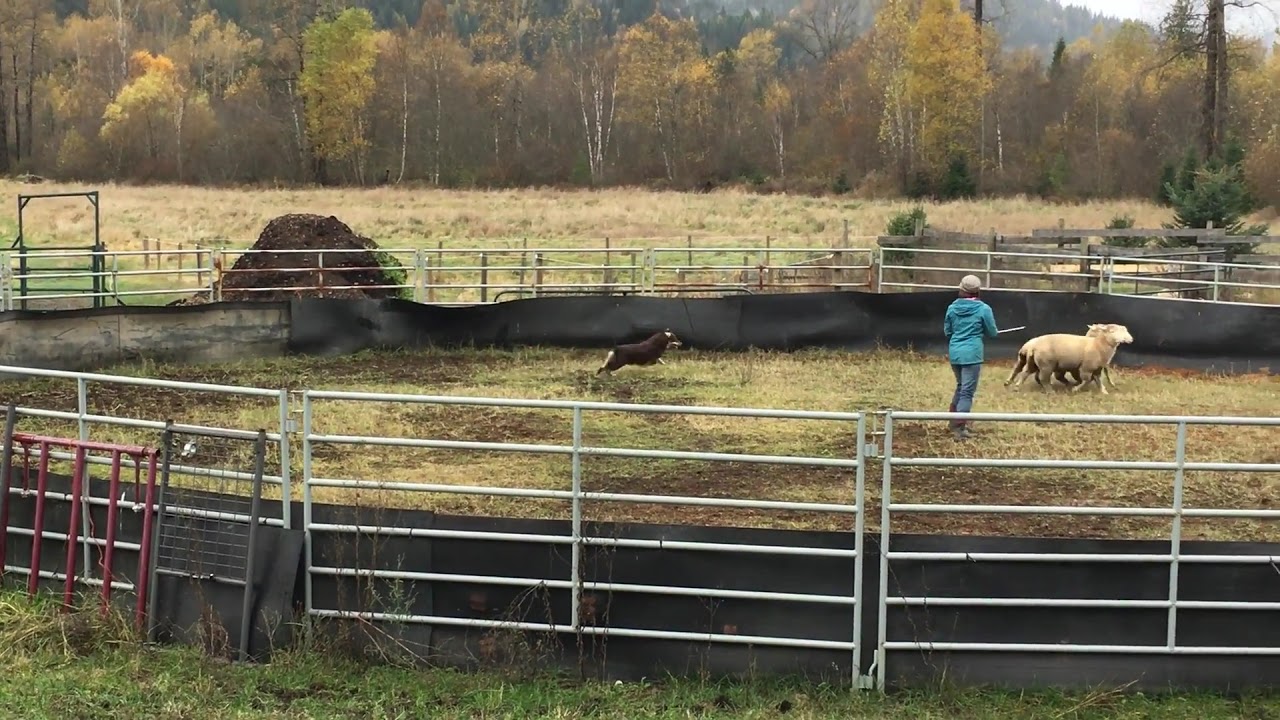The image showcases a scene on a farm with a metal, circular pen outlined by silver fences partially covered at the base with black fabric. Inside the pen, a woman dressed in a blue hoodie, blue jeans, and a white hat is seen engaging with the animals, possibly training or herding two sheep. A black herding dog with brown markings on its snout, tail, and feet aids her from the left side of the pen. The ground within the pen is a mix of tan, sparse grass with patches of exposed dark brown soil. In the background, there is an expansive view of a rural landscape, featuring trees in various shades of green, yellow, and brown, highlighting a serene fall setting. The image lacks any visible barns or houses, maintaining a focus on the fenced enclosure and its inhabitants.